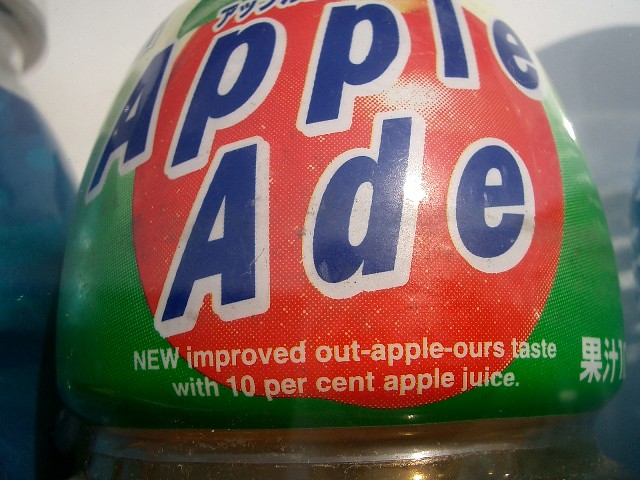This close-up image of a juice bottle showcases a vibrant and colorful label dominated by shades of green, orange, navy blue, and white. The label prominently displays the product name, "Apple Aid," in large, bold blue letters outlined in white, giving it a 3D effect. Underneath "Apple Aid," the label highlights "Apple" again, emphasizing its primary flavor. Notably, the orange circle is accented further with phrases like "New Improved Out-Apple-Hours Taste" and "10% apple juice" written in white on a green base. The label also features some Asian characters, possibly Korean, Japanese, or Chinese, at both the top and bottom. In the background, additional bottles can be seen, including a partially visible blue bottle to the left and a possible pink bottle to the right, adding depth and context to the image.